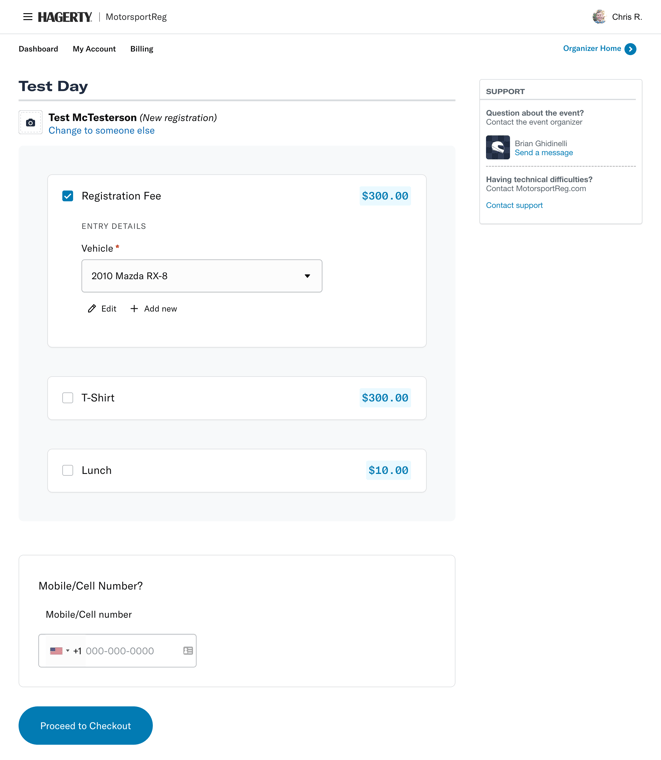This image showcases a section of the Hagerty website centered around motorsport activities. In the top right corner, there's a profile section featuring the name Chris R and a profile picture. Just below, on the left, are navigation options labeled "Dashboard," "My Account," and "Billing." On the right side underneath the profile, it says "Organizer Home" next to a blue button.

Moving further down, the left side of the page highlights a section labeled "Test Day" which features a light grey box. This box includes a camera icon and information about a test registration under the name "Test McTesterson." Key details include:
- Registration Change: Option to change the registration to someone else.
- Registration Fee: $300
- Entry Details: Vehicle listed is a 2010 Mazda RX-8.
- T-shirt Option: Available for an additional $300, selectable via a checkbox.
- Lunch Option: Available for an additional $10, selectable via a checkbox.

At the very bottom of the grey box, there is a field to enter a mobile or cell phone number, followed by a "Proceed to Checkout" blue button. To assist users, a support section is visible in the top right corner.